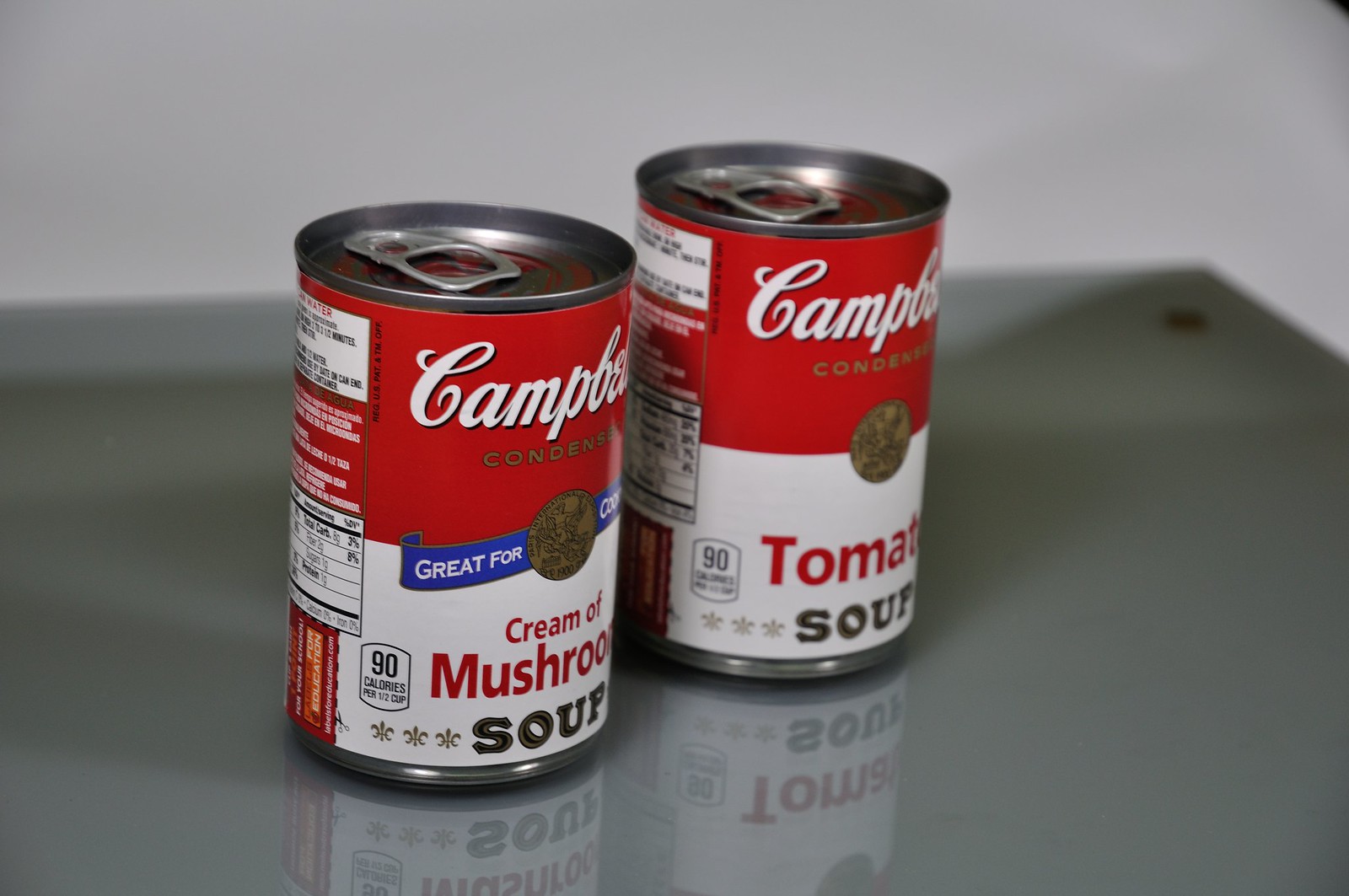This photograph captures two iconic cans of Campbell's soup prominently displayed in the center of a smooth, gray metal or plastic surface. The reflective nature of the surface allows for a clear reflection of the cans below them. The backdrop features a blurred, stark white wall with a hint of black in the upper right-hand corner, suggesting an object just out of frame.

The two cans are slightly angled towards each other, creating a balanced composition. The can on the left is Campbell's Cream of Mushroom Soup, notable for its red and white label, with a touch of blue and a bold statement near the logo that reads "Great for Cooking." The can on the right is Campbell's Tomato Soup, also featuring the classic red and white design.

Details of the nutritional information and ingredients lists are partially visible on both cans. In the lower right corner of the surface, there's a small black dot, potentially a screw or rivet, adding a subtle point of interest. The high-contrast background and reflective surface ensure that the viewer's attention remains focused on the two iconic soup cans.